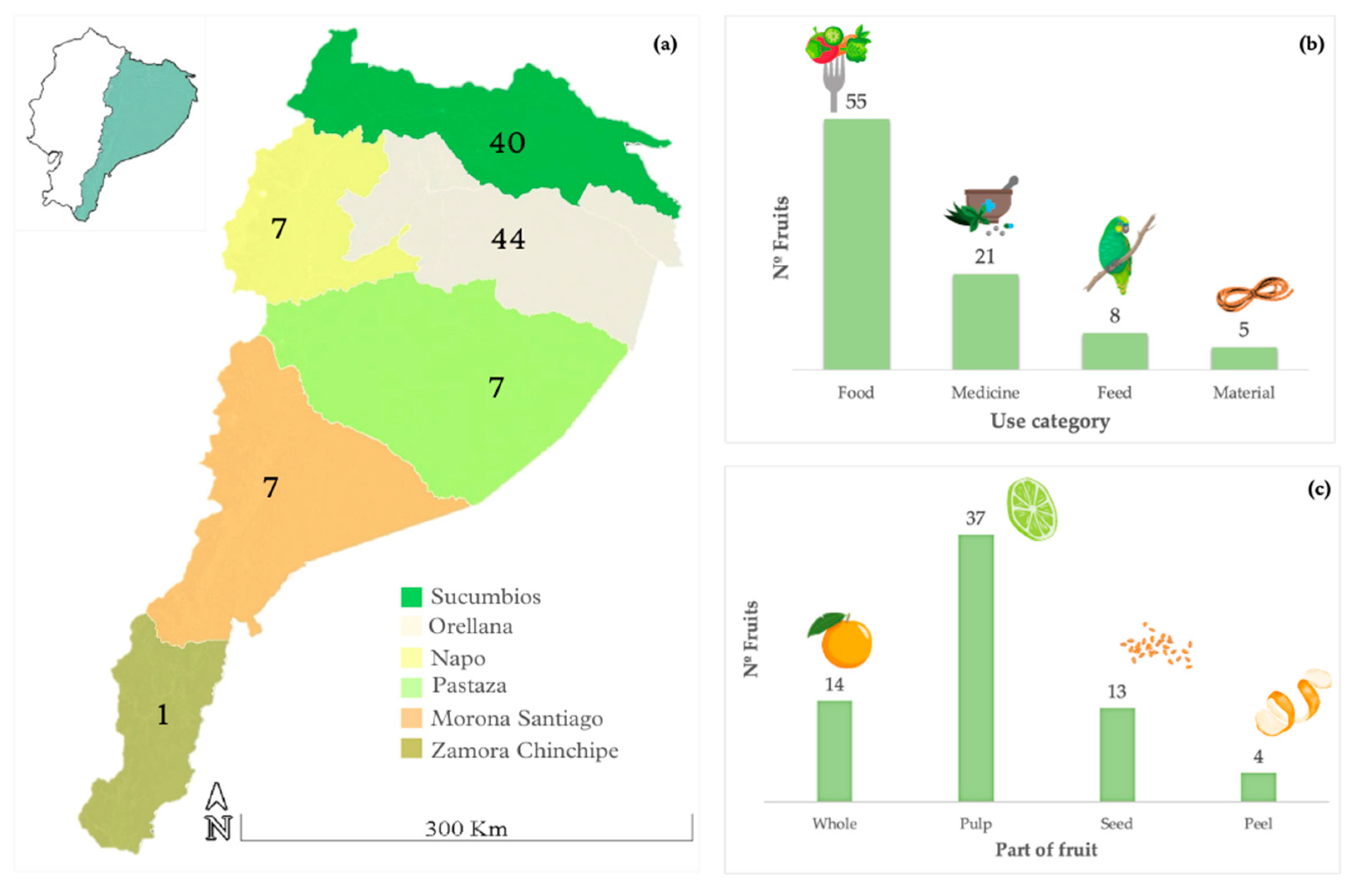The image in question is slightly wider than it is tall and resembles a slide rather than a traditional textbook page. On the left side, there is a map structured like a peninsula and divided into different color-coded sections—light green, dark green, off-white, yellow, orange, and brown. Each section is numbered and has corresponding labels situated below the map. The names in these labels include terms such as succumbios and oreana. A key is provided to explain the color meanings.

On the right side of the image, there are two graphs labeled A and B. Graph A categorizes fruits based on their uses: the highest being for food, followed by medicine, feed, and material. Graph B breaks down parts of the fruit into whole, pulp, seed, and peel, showing quantities of 14 for whole, 37 for pulp, 13 for seed, and 4 for peel. This detailed depiction appears to be a visual presentation of data related to a specific landmass and the various uses and parts of fruits within that region.